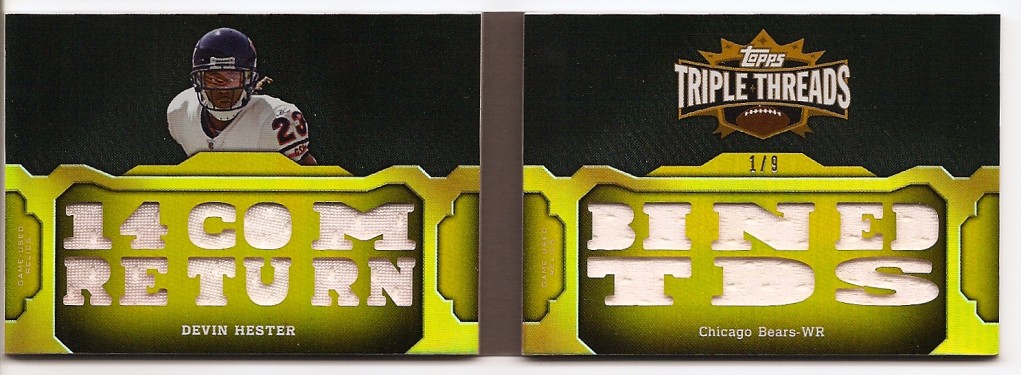The digital image depicts a Topps Triple Threads sports card featuring Devin Hester of the Chicago Bears. The card displays two almost identical images side-by-side, each showing Hester in a white jersey with the number 23 and a black helmet. The background is predominantly black, transitioning to a yellow ornate pattern resembling a fence at the bottom.

On the left side of the card, the text reads "14 COM. RETURN, DEVIN HESTER" in white, diamond-like lettering. The yellow bottom edge features a fancy design. The right side mirrors the left but with additional details, including the "Topps Triple Threads" logo in white capital letters and a small football icon at the top. In the yellow section below, it reads "1 OUT OF 9" and "BINED TDS" in capital letters, with "Chicago Bears W-R" in smaller font.

The image appears to be a digital representation rather than a printed card, created by the sports card company Topps.